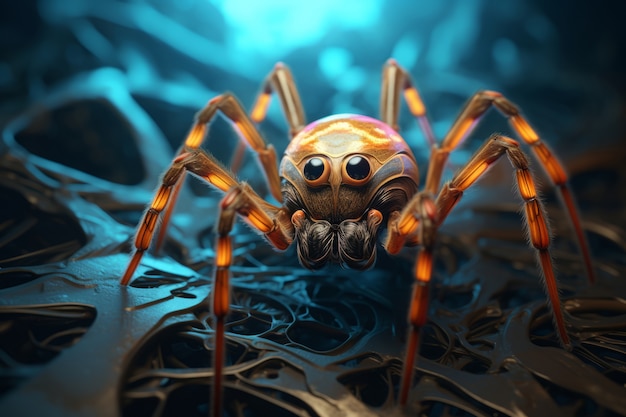An exquisite, computer-generated spider dominates the center of this image, standing on a complex, tangled structure of woven metallic pieces with numerous holes. The background is an abstract blur of dark teal and black, evoking a digital or illuminated scene. The spider's eight legs are adorned with bands of glowing oranges, browns, and reds, giving it a vivid, almost ethereal appearance. Its body exhibits a mix of pink, yellow, and orange hues, with striking black eyes outlined in an orangish hue, fixating directly at the observer. Though the fangs are not clearly visible, there's a noticeable black area where they should be, suggesting an imminent jump.